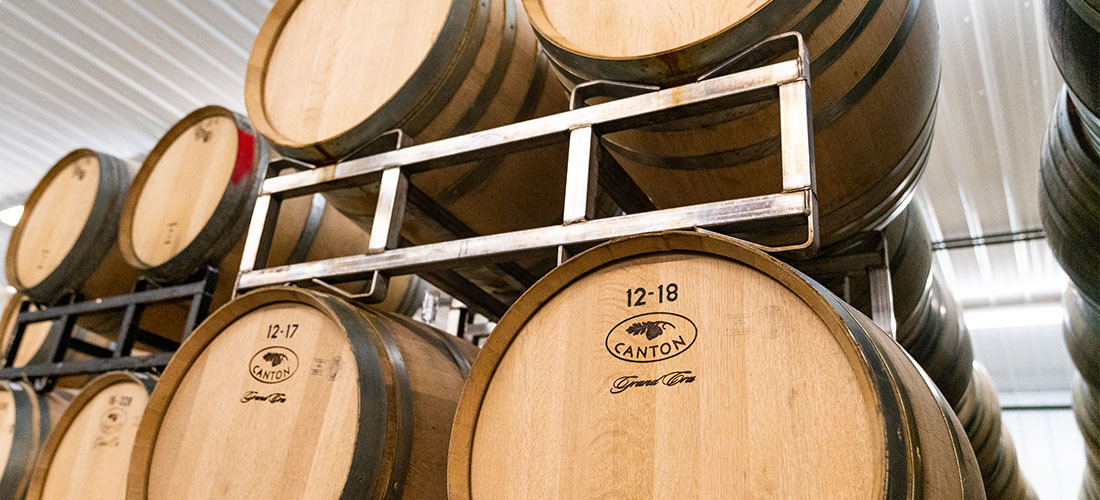This photograph captures a spacious warehouse filled with numerous light brown wooden wine barrels, meticulously organized in rows and stacked on metal frames of both black and chrome steel. The barrels are arranged in two prominent layers, each row extending all the way to the back, with estimates of ten barrels per row horizontally, and four vertically. These barrels display a consistent labeling system: each has a label on top with numbers such as 12-17 and 12-18. Below this numbering, a logo featuring a grape leaf is visible, under which the word "Canton" is prominently displayed. It's difficult to decipher the smaller text beneath "Canton" due to its size, but a signature in black is also present. The warehouse itself has a white ceiling, likely made from corrugated metal, creating an organized yet industrial atmosphere. Fluorescent-like lights illuminate the storage area, highlighting the rows and the intricate details on each barrel.